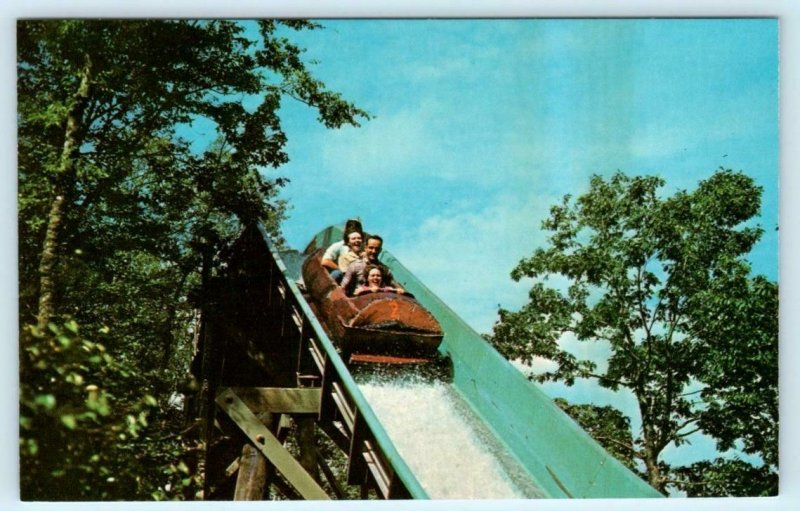This vintage photograph, enclosed in a light blue border, captures a memorable moment on Disneyland's Splash Mountain ride. The faded image depicts a family of four in a hollowed-out log flume as it plunges down a steep, blue-water slide supported by large, light brown beams. The front seats a small child, followed by a man, then a woman, and another man at the back. The expressions on their faces, a mix of smiles and laughter, capture the thrill of the ride. Surrounding the flume are tall trees with vibrant green leaves, and the scene is set against a light blue sky scattered with a few white clouds, adding to the scenic backdrop of their adventure.